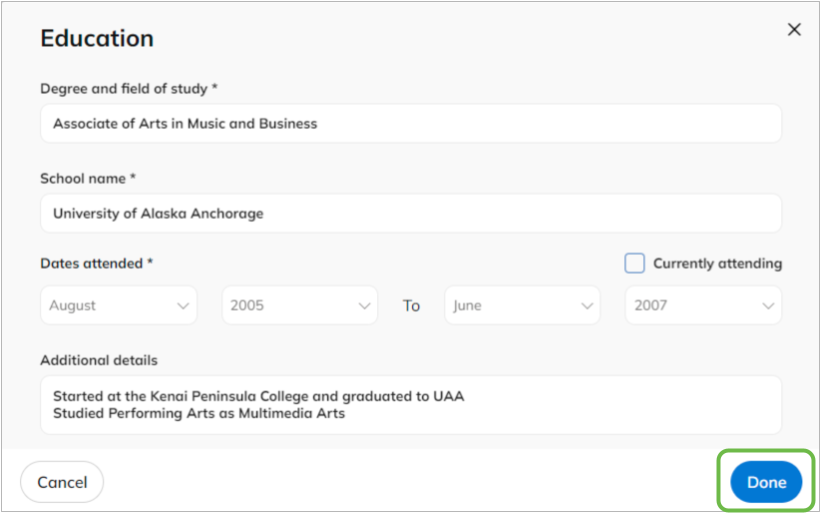A detailed screen capture from an application platform, showcasing an 'Education' section prominently at the top. The content lists the details of an individual's academic background, featuring the following fields: 

- **Degree & Field of Study:** Associate of Arts in Music and Business
- **School Name:** University of Alaska Anchorage
- **Dates Attended:** August 2005 to June 2007
- **Additional Details:** Started at Kenai Peninsula College and graduated from UAA, studied Performing Arts as well as Multimedia Arts.

The interface appears to be part of a job search website or a professional networking platform. At the bottom of the section, there are two navigational buttons: a 'Cancel' button for reverting changes, and a 'Done' button highlighted in blue with white lettering for saving the information. A green box has been manually drawn around the 'Done' button, presumably to draw attention to it.